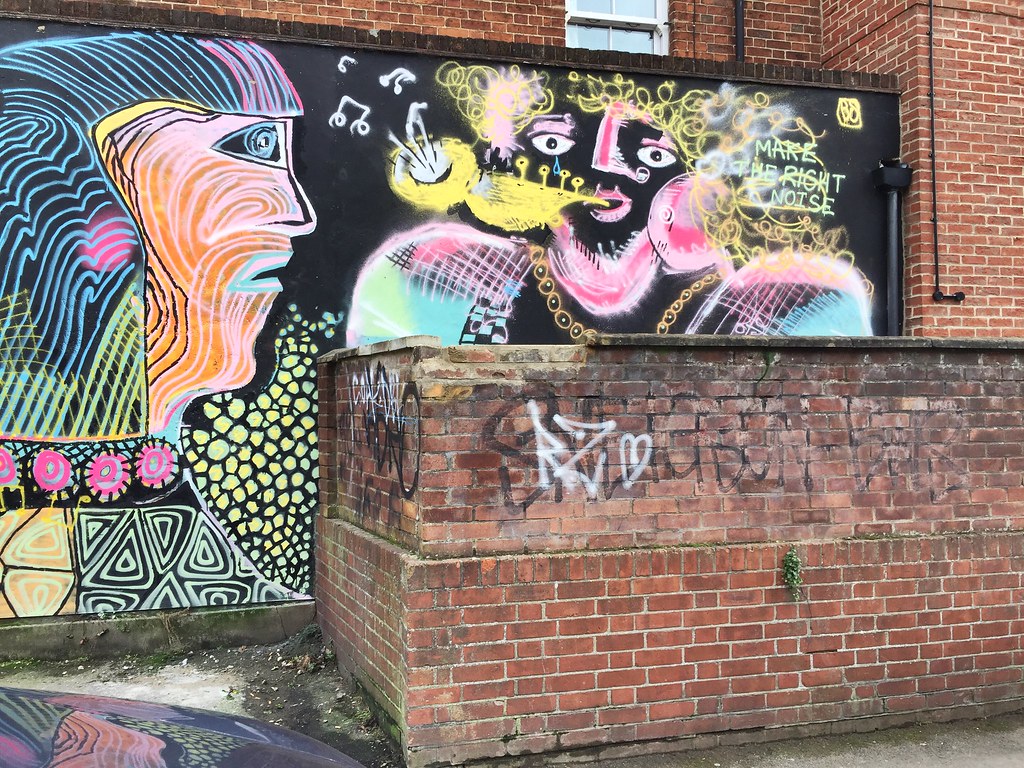The photograph captures a mural featuring a striking, colorful artwork on an aged, red brick building. The mural, set against a black painted background, utilizes a style resembling chalk art due to its blurred edges. The central figure is a person with curly yellow hair, playing a stylized gold instrument, likely a trumpet or a saxophone, with vibrant music notes emanating from it. The figure is adorned in a vividly colorful outfit of pinks and blues, and their curly hair inscribes the phrase "Make the Right Noise."

Adjacent to this musician is another uniquely stylized figure facing them, characterized by Aztec-like features. This figure has an orange face with swirling patterns, blue eyes, and multi-colored wavy hair in shades of blue, pink, and yellow. They wear a beaded necklace with pink circles and a garment decorated with intricate triangular patterns. The entire scene is replete with dynamic elements such as trippy black and white triangles and small yellow spots, contributing to the mural's overall whimsical and vibrant aesthetic. The lower wall of the structure also features additional graffiti, including letters and symbols, further adding to the urban artistic tapestry.